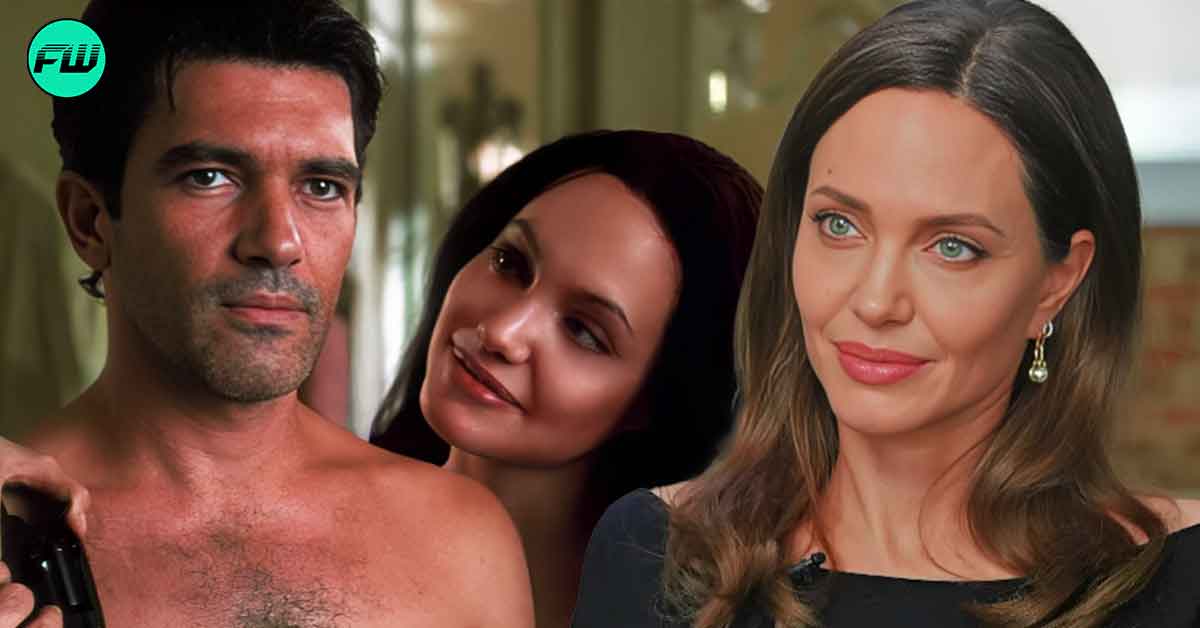This horizontally aligned rectangular image features a combination of two distinct pictures. On the left side, a younger Antonio Banderas is depicted shirtless, facing the camera from his chest up with his short black hair and looking into a mirror. Next to him is an unidentified actress in the middle with long, straight black hair, smiling up at him over his shoulder. Standing to the right of Banderas is Angelina Jolie, who is captured looking off into the distance with a big smile, showcasing her long wavy brown hair, green eyes, drop earrings, and pink lipstick. Overlaying part of this background scene on the right half of the image is another cutout of Angelina Jolie. In this cutout, she is wearing a black dress with a small microphone clipped to the collar, and pearl earrings are visible on both ears. Her hair flows past her shoulders, and her bluish-green eyes gaze ahead, adding a layered effect to the composition. The backdrop appears to represent the interior of a home or building, depicted in a slightly blurry manner. Additionally, a green circular logo with a black border and the letters "FW" inside is positioned in the upper left corner of the image.